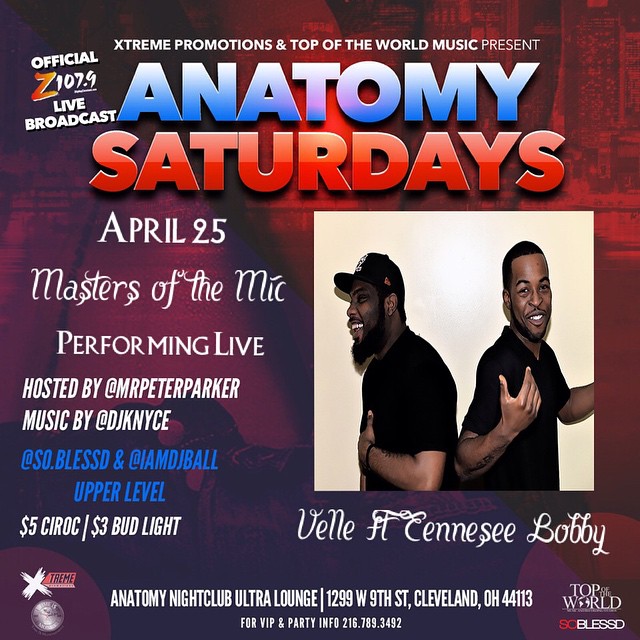The poster features a vibrant background predominantly in purple and red, advertising a special event hosted by Z107.9. At the top left corner, the poster proudly declares it as an official Z107.9 live broadcast. In white text at the top center, it reads, "Xtreme Promotions and Top of the World Music present: Anatomy Saturdays." Prominently displayed is "April 25th Master of the Mic Performance Live," hosted by @MrPeterParker with music by @DJKNYCE. 

To the right, there is an image of two men, both wearing black short-sleeve shirts, facing each other—one facing left and the other facing right, with the latter staring directly ahead. 

Additional text reveals the event details: "Performing live with music by @SoBlessed and @IAmDJBball." The venue, Anatomy Night Club Ultra Lounge, is located at 1299 West 9th Street, Cleveland, Ohio, 44113. Ticket prices are mentioned as $5 for a rock and $3 for a Bud Light, with VIP and party information available at 216-789-3492.